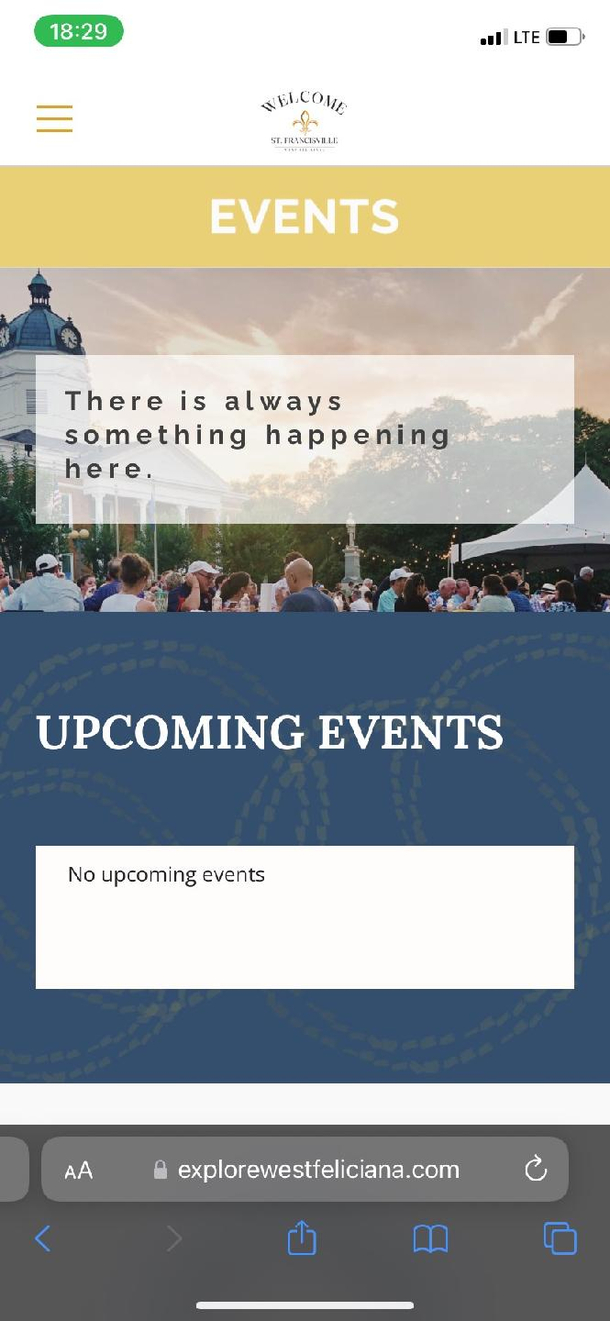The image is a screenshot from an iPhone screen captured at 6:29 PM, displaying a website dedicated to events. The iPhone shows a strong signal and a battery level at approximately 55%. The screenshot features a website with a prominent heading at the top that reads "WELCOME" in capital black letters, accompanied by a small fleur-de-lis symbol below it.

Beneath this heading is a rectangular box with a tannish gold background and white capital letters spelling "EVENTS." Below this banner is a photograph depicting a crowd of people outdoors, standing near a tent and a significant building with a prominent roof that resembles the architectural style of a capitol or possibly the White House.

Embedded within the image, there's a white box containing the phrase "There’s always something happening here." Further down, a section with a blue and gold background features the text "Upcoming Events" in white capital letters. However, a black-lettered box within this section states "No upcoming events."

At the very top of the screenshot, the toolbar includes the URL "explorewestsaliciana.com" along with various menu buttons.